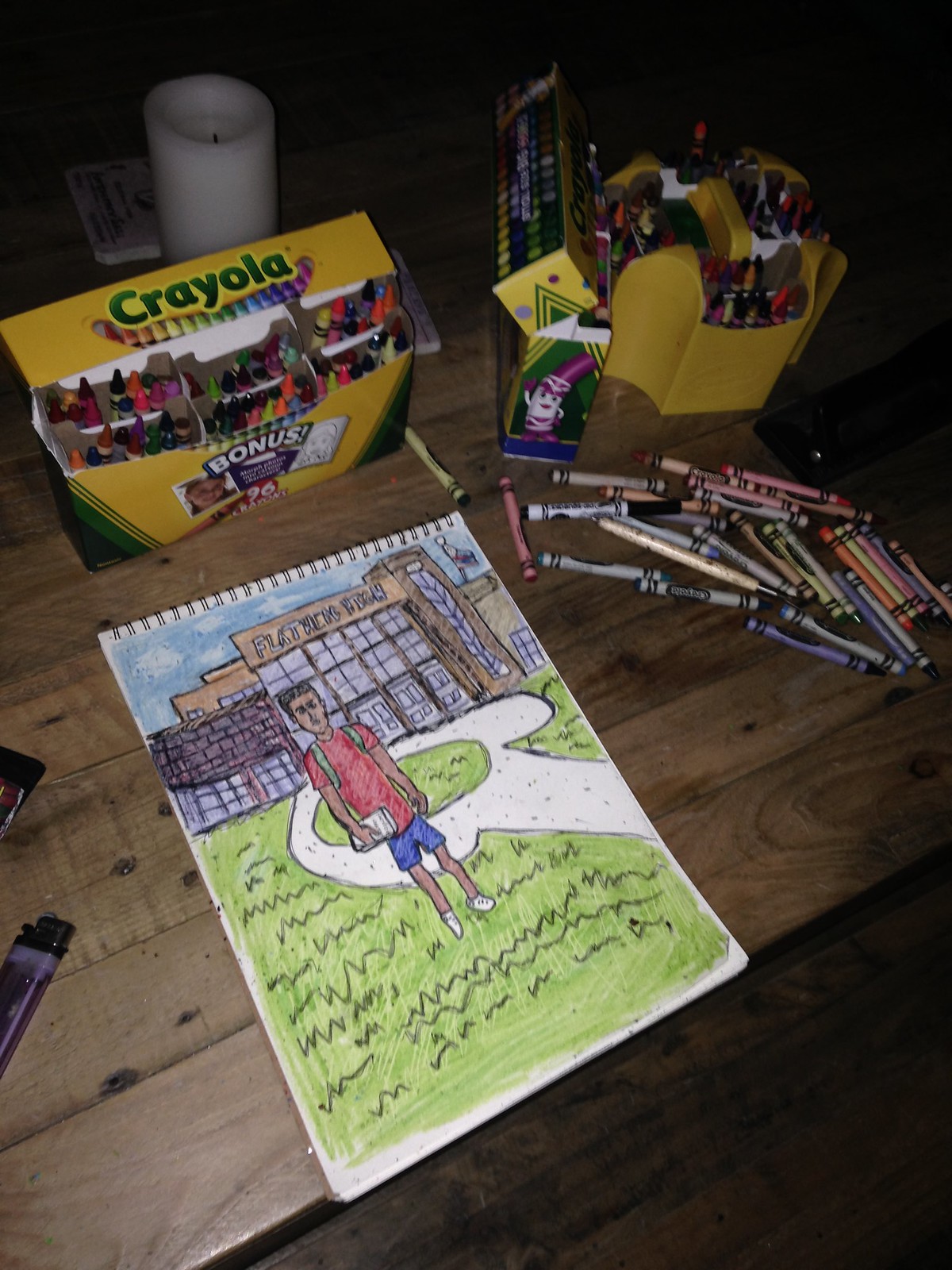The image is a detailed, angled view looking down at a large spiral sketch notebook resting on a medium to dark brown wooden table. The open notebook contains a vibrant crayon drawing of a boy wearing a red t-shirt, blue shorts, and white shoes, with straps of a green backpack visible, as he stands on a green grassy area. He holds books in his left hand and is positioned in front of a large brown brick school building with multiple tall windows. A light-colored walkway, dotted with black spots, curves in a circle in front of the school. Surrounding the notepad on the table are various art supplies: loose crayons to the left, two boxes of Crayola crayons at the top—one a recognizable yellow and green box—and a round yellow crayon holder in the top right, filled with various crayons and writing tools. Additionally, a purple lighter with a black top peeks into the frame from the bottom left, and a tall white candle stands behind one of the Crayola boxes, adding an extra layer of detail to the scene.